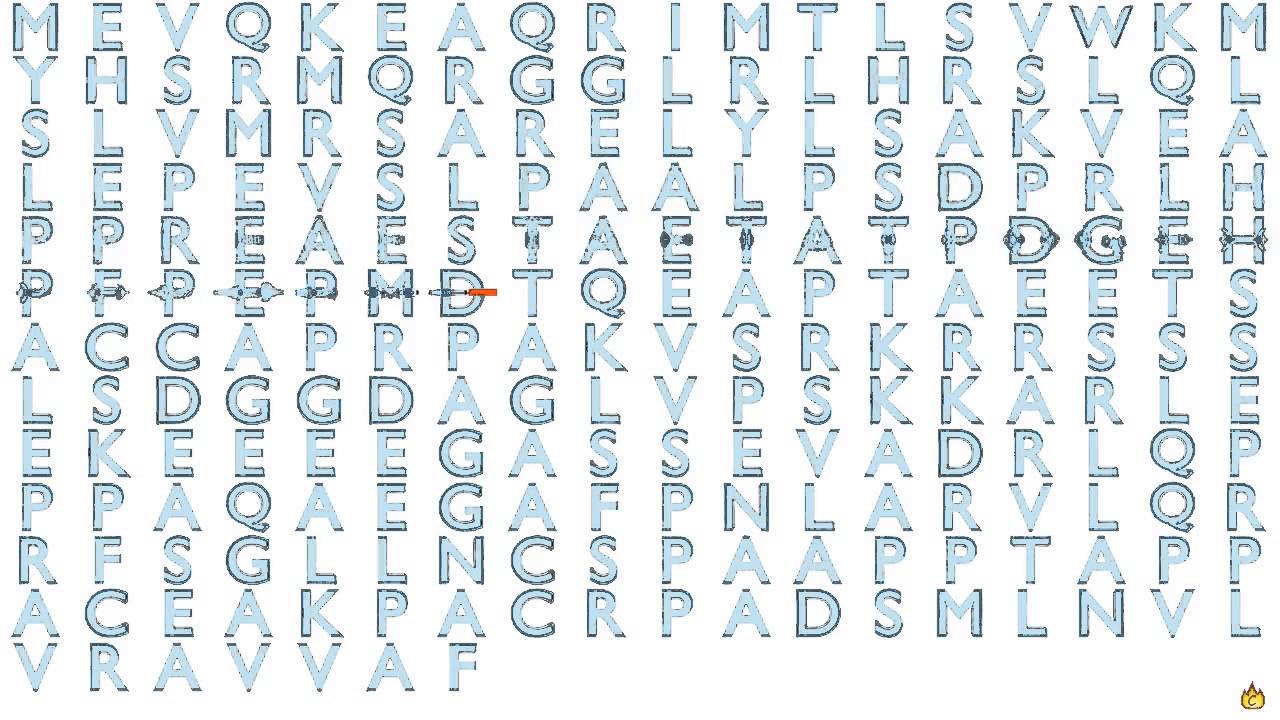This image is a screenshot from the game "Piercey Bee," showcasing a grid of randomly arranged capital letters. The letters, uniformly light blue with thin black borders, are organized into 13 distinct rows. Rows 4 and 5 feature stylized variations of certain letters, decorated with additional designs while maintaining their original shapes. The collection of letters appears to be randomly assorted, without forming any recognizable words. In the bottom right corner, there is a small yellow flame symbol containing the capital letter "C."